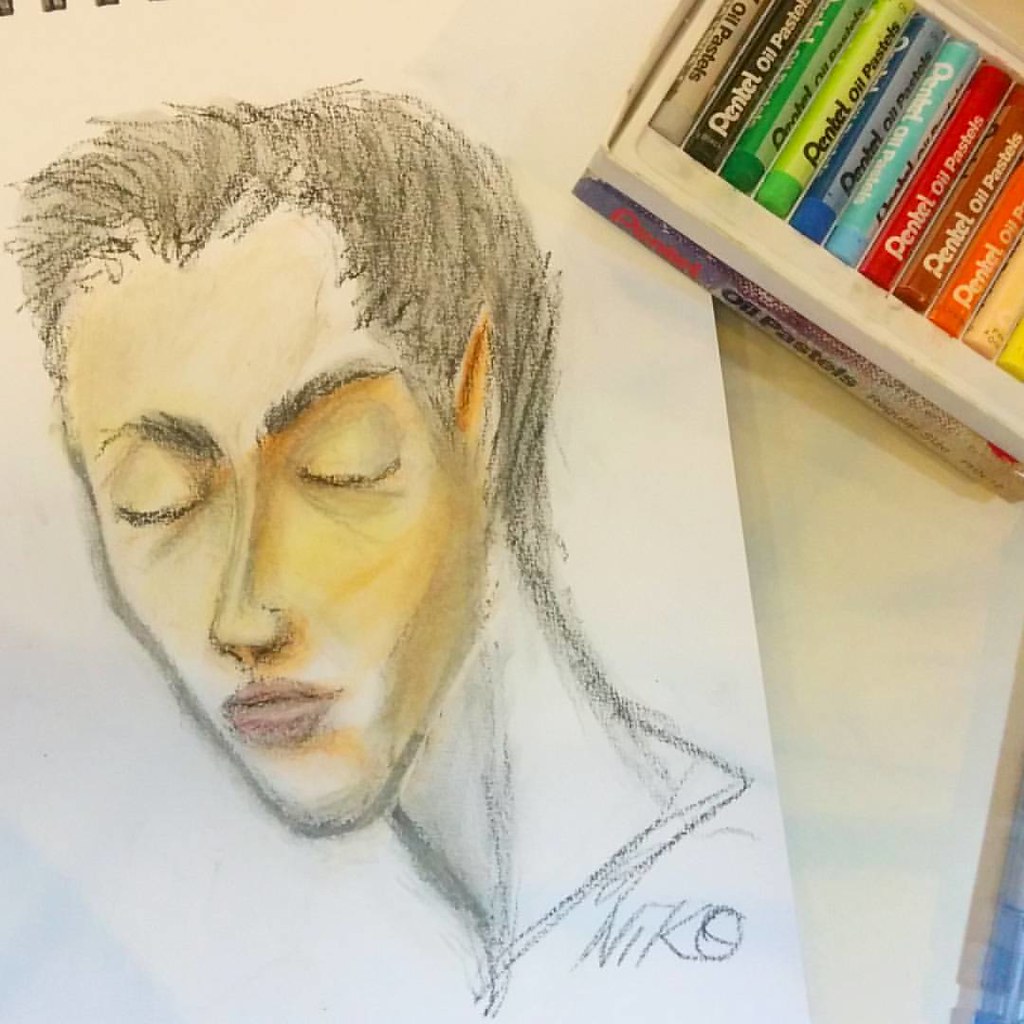This image captures a top-down view of a drawing on a white piece of paper, likely from a spiral-bound notebook, as evidenced by the visible edges of the spiral at the very top left. The artwork, seemingly created with Pentel oil pastels, portrays a man's face with his head turned towards his left shoulder but facing more directly towards the camera. His eyes are closed, and he features high arched eyebrows, short dark hair with no part line, and a long, angular face with a prominent V-shaped jaw and chin, a pronounced nose, and thick lips.

The sketch is predominantly in black and white, with black lines outlining his hair, face, eyebrows, eyelashes, and neck. His face is shaded with yellow, his pointy left ear filled in with an orangish-red color, and a slight pink tint applied to his lips. There's also a striking aqua line accentuating his nose. The relaxed, slightly pursed expression and the detailed shading give depth to the portrait. The drawing is signed "N-I-K-O" under the neck on the bottom right. The upper right corner of the image reveals a box of Pentel oil pastels laid horizontally, showing a variety of at least 10 to 12 colors, hinting at the artistic tools used to bring this vivid portrait to life.